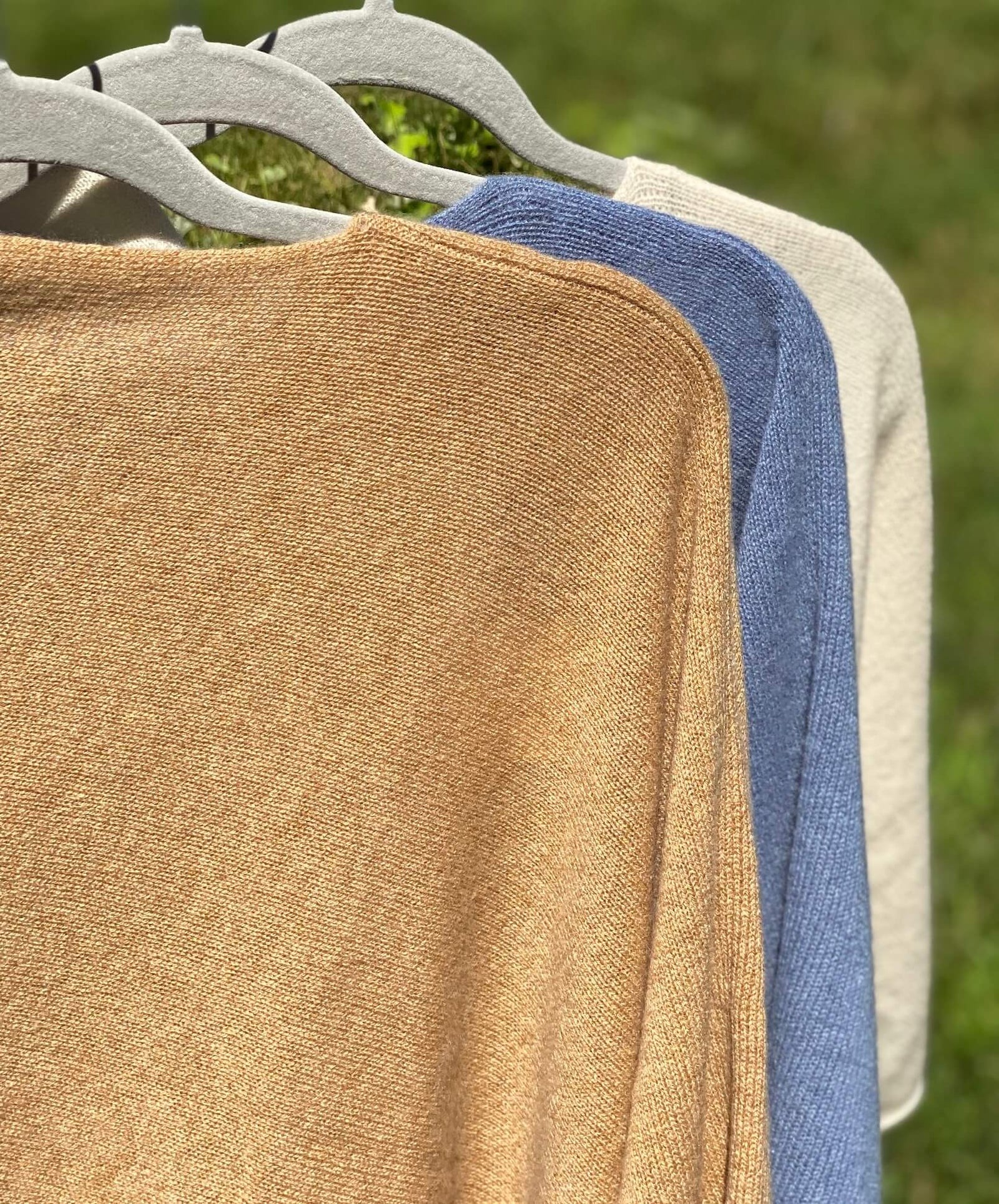In this image, three sweaters are hanging side by side on a soft, white, spongy hanger with round edges, though the hooks of the hangers are not visible. Each sweater is made of a knit material. The first sweater in the front is a honey-gold beige knit fabric, the middle one is blue, and the one at the back is an off-white cream color. The right sleeve of the sweaters is visible while the left side is cropped out of the image. The background is a blurred, faded gray with out-of-focus green elements that resemble plants or trees, giving the impression that the clothing might be hanging outdoors. The sweaters dominate the frame and are very plain, without any design or pattern, extending towards the left side of the image.